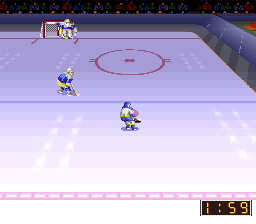This image is a nostalgic screenshot capturing a moment from a vintage video game set in an ice hockey arena. The scene centers around a meticulously detailed ice rink, complete with lines and zones specific to a hockey court. Three pixelated characters animate the scene: one is positioned in the center, presumably the player's character, with another character standing slightly above and to the left, suggesting an opposing defender. In the top left corner, a goal post is visible, guarded by a pixelated goalie, characteristic of the game's era. In the bottom right corner, a timer ticks down, showing 1 minute and 59 seconds remaining in the game, adding a sense of urgency and excitement to this classic sporting moment.